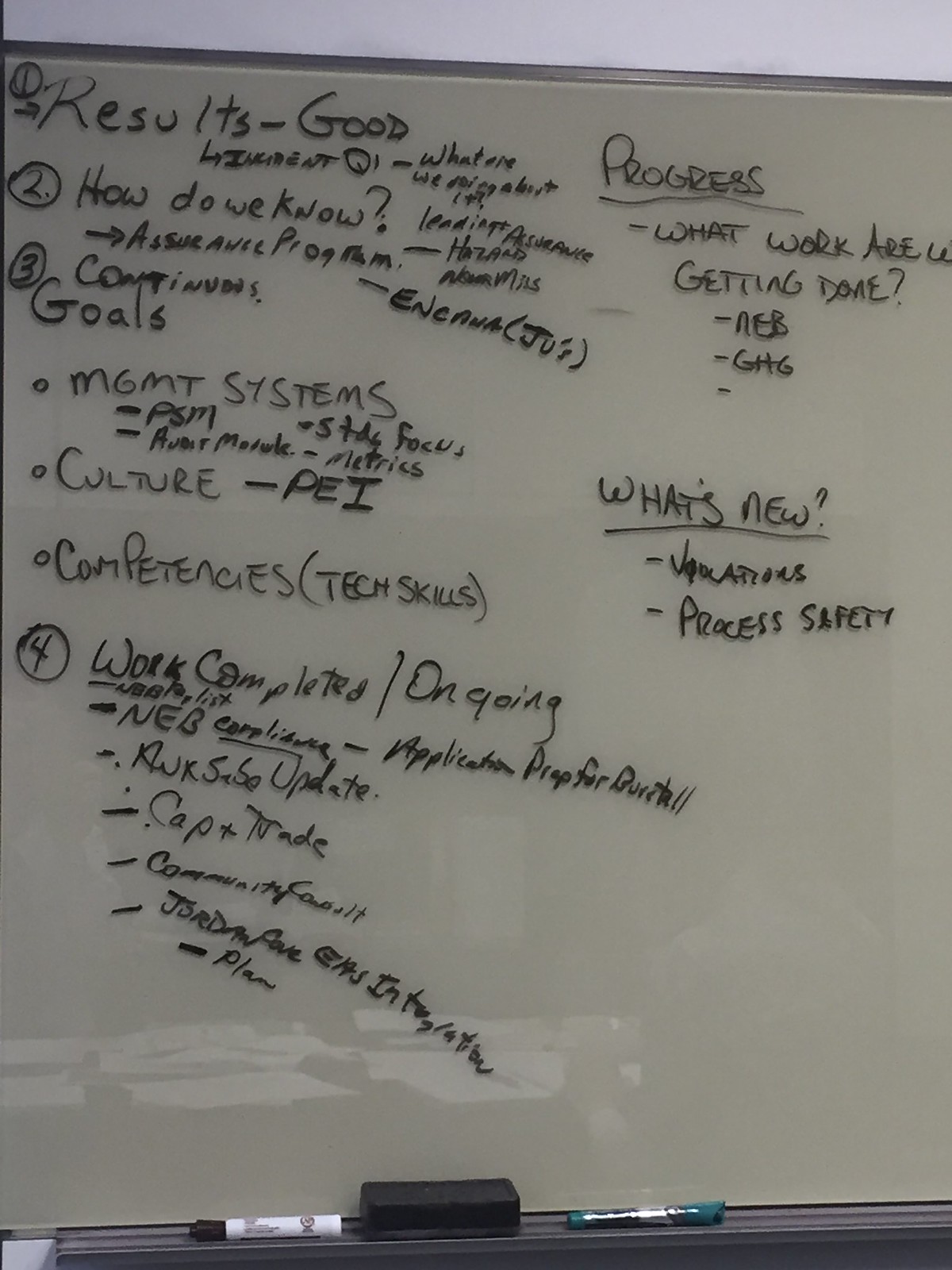The image is of a whiteboard, possibly located in a classroom or business meeting room. The whiteboard has extensive black writing on it, organized into a numbered list on the left side. The top of the whiteboard starts with "1. Results - good," followed by additional less legible text. The second item is circled and asks, "How do we know?" with a note about an "Assurance Program" below it. Item three lists "Continues goals" followed by a bullet point list including "Management systems," "PSM," "Study focus," "Metrics," "Culture - PEI," and "Competencies." The fourth item reads "Work completed/ongoing," accompanied by several sub-bullet points. On the right side of the whiteboard, the words "Progress" and "What's new" are underlined. At the bottom of the whiteboard is a ledge holding two dry erase markers and an eraser between them. The backdrop includes part of a gray ceiling or wall and hints of a window or door's reflection, suggesting the presence of people or a class setting.